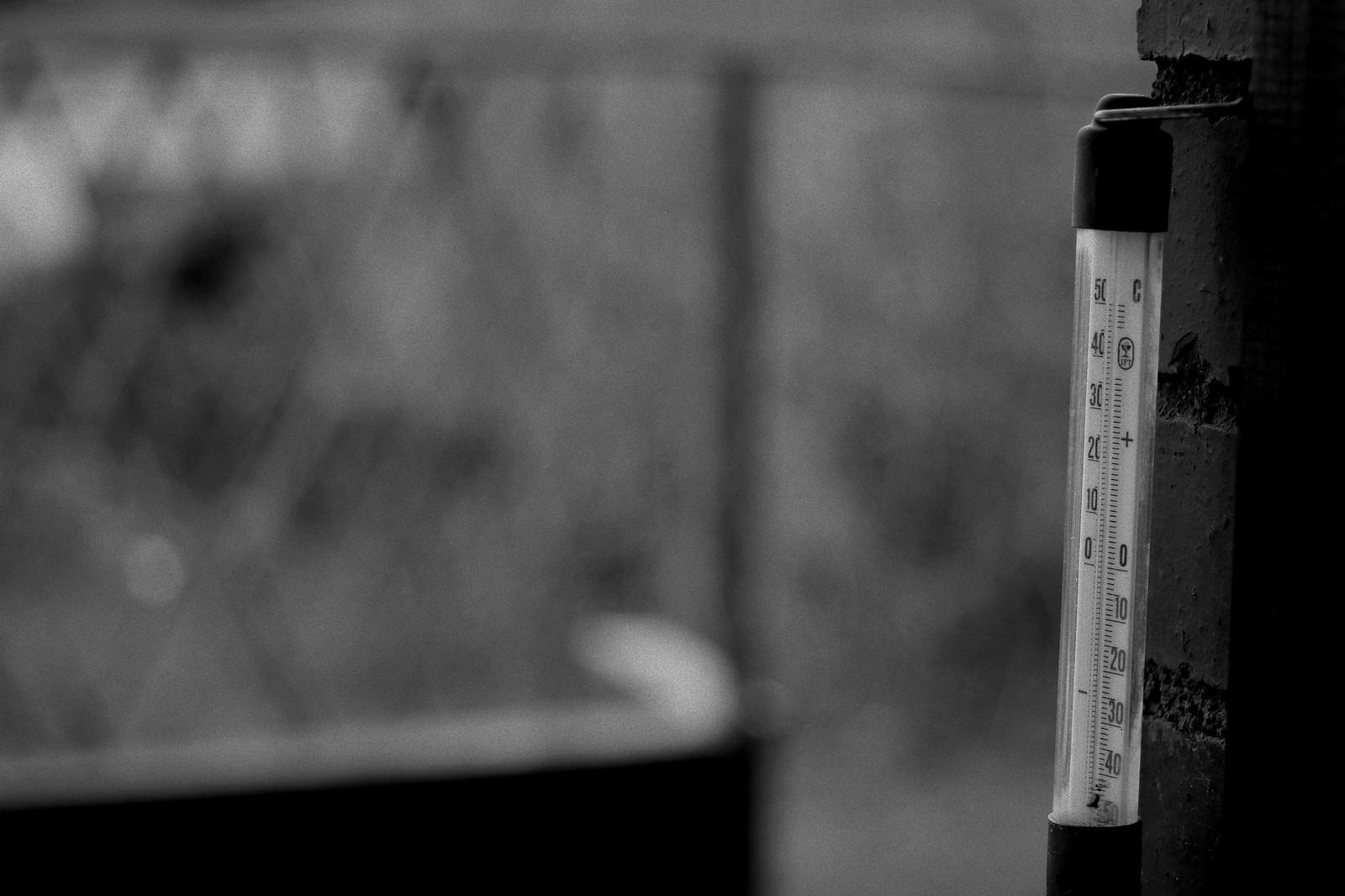A captivating, smoky black and white photograph captures an outdoor scene shrouded with shadows. The image features a blurry depiction of part of a wooden structure, which adds to the mysterious ambiance. Attached to the right side of the wooden structure hangs a thermometer, fastened securely with a metal hook. The thermometer is marked with black numbers, including 50, 40, 30, 20, 10, and 0 degrees Celsius, along with intricate black line markings. Despite the dim lighting, the thermometer's measurements and the capital letter 'C' plus sign are discernible, adding a tangible focal point to the hazy surroundings.